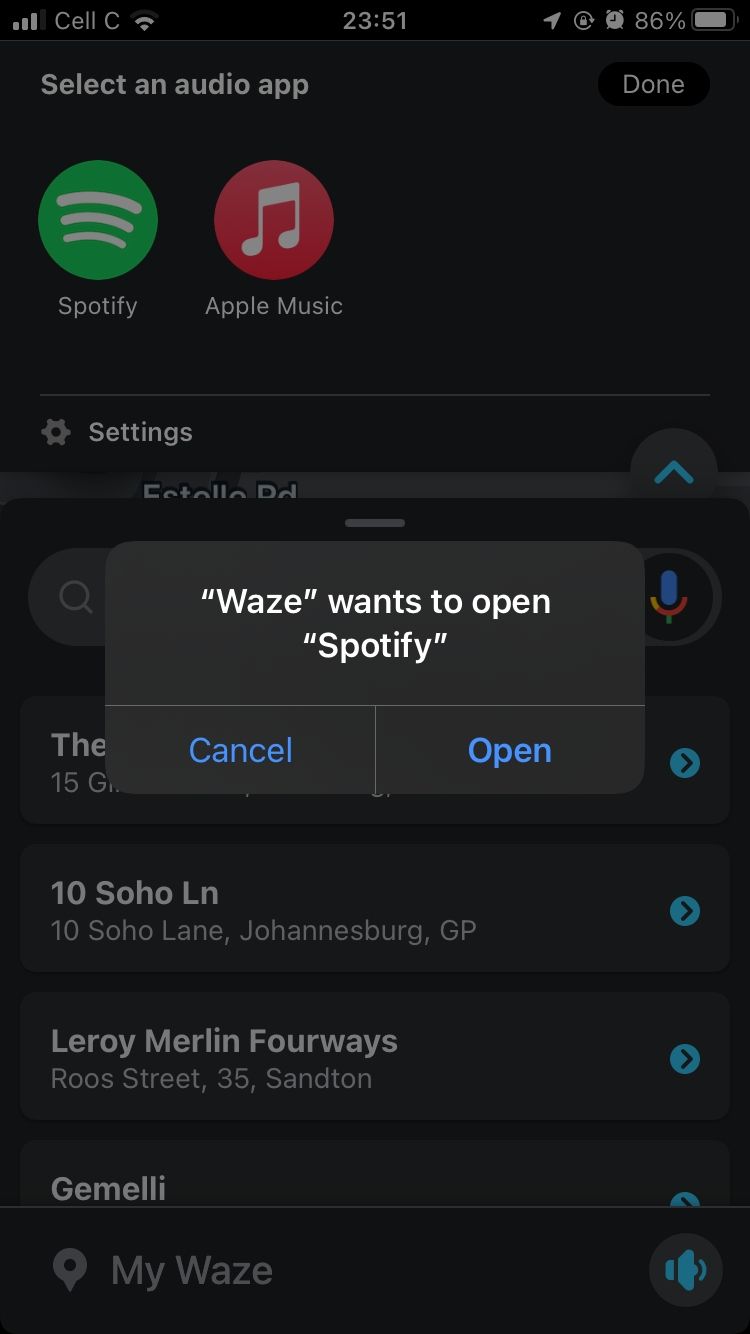This image is a screenshot taken from an iPhone, displaying an interface where the Spotify app is involved. The background of the page is black. At the top left, there's a text header saying "Select an audio app." On the top right, a button labeled "Done" is visible.

Beneath this, there are two prominent logos: the Spotify logo, which is a green circle with three white, curved lines in the center, and the Apple Music logo, a red circle with a white music note emblem inside it.

Further down the screen, there's a section labeled "Settings," followed by a pop-up alert. This alert, originating from the navigation app Waze, reads "Waze wants to open Spotify." It provides two action buttons: "Cancel" and "Open," allowing the user to either cancel the action or proceed to open Spotify.

At the bottom of the screenshot, there is a "My Waze" section, accompanied by a speaker icon to the right.